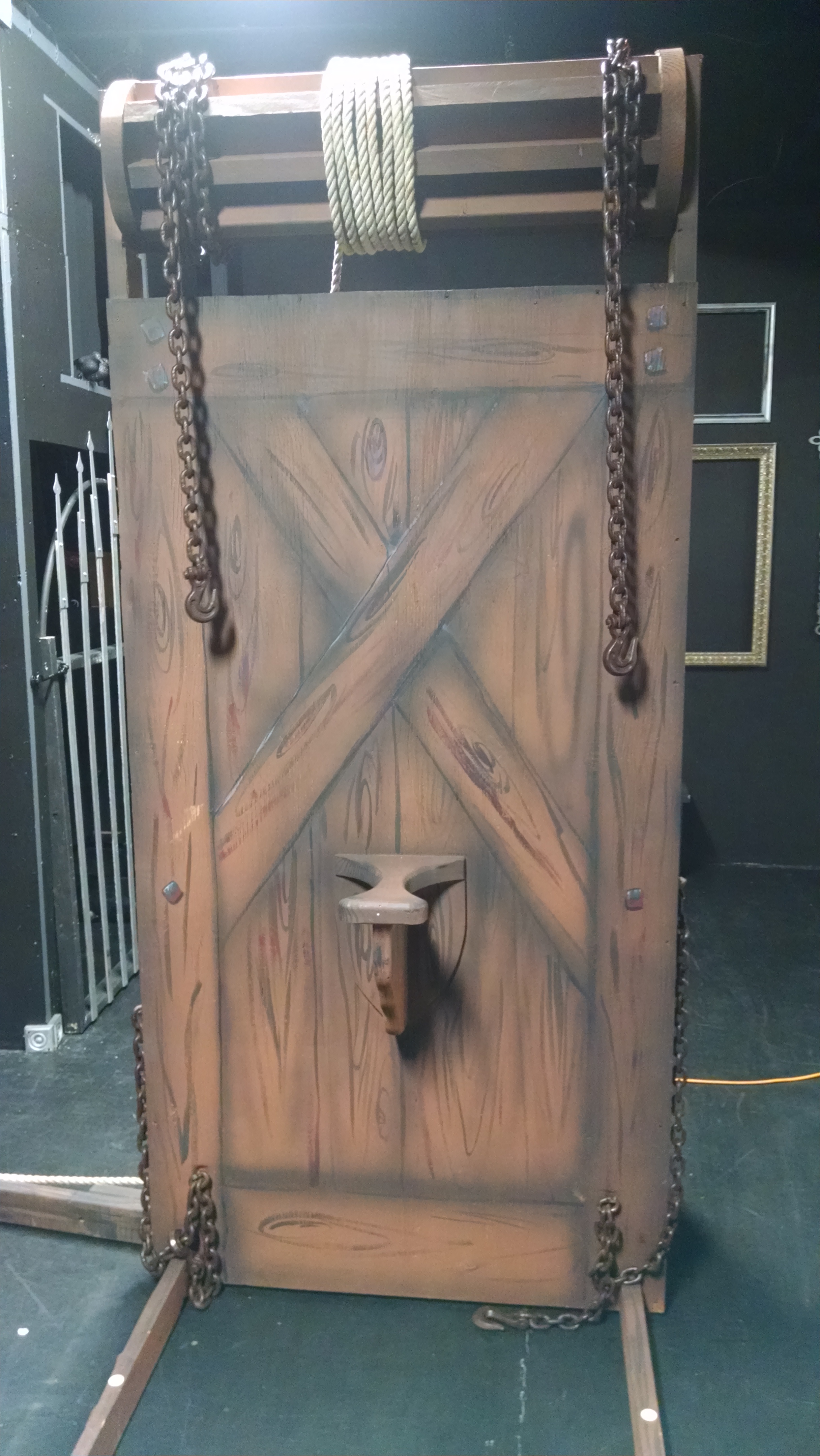The image depicts an ominous scene centered around a puzzling apparatus that resembles a dark brown wooden door with diagonal wooden slats and a horizontal crosspiece. Attached in the middle is a thin, protruding ledge, giving the impression that it serves as a sort of seat. The door-like structure itself is mounted on a brown metal stand, which is not connected to any walls but stands independently within a dark room. Heavy-duty chains hang from the top of the structure, with a revolving spiral mechanism adorned with white rope and additional chains wrapped around it. These chains appear to be designed to wrap around or unwind from the device, suggesting a mechanism for manipulation.

The overall ambiance is eerie, given the black walls and floor, and the background features a doorway with a spiked silver fence, heightening the sinister atmosphere and suggesting an adjoining, equally unsettling chamber. The apparatus evokes strong imagery of a medieval torture device, possibly designed to restrain someone seated on the central ledge while the chains from the top and bottom secure them. The turning mechanism at the top implies a function to stretch the individual restrained on the device, further supporting the notion of it being a device for inflicting physical torment.